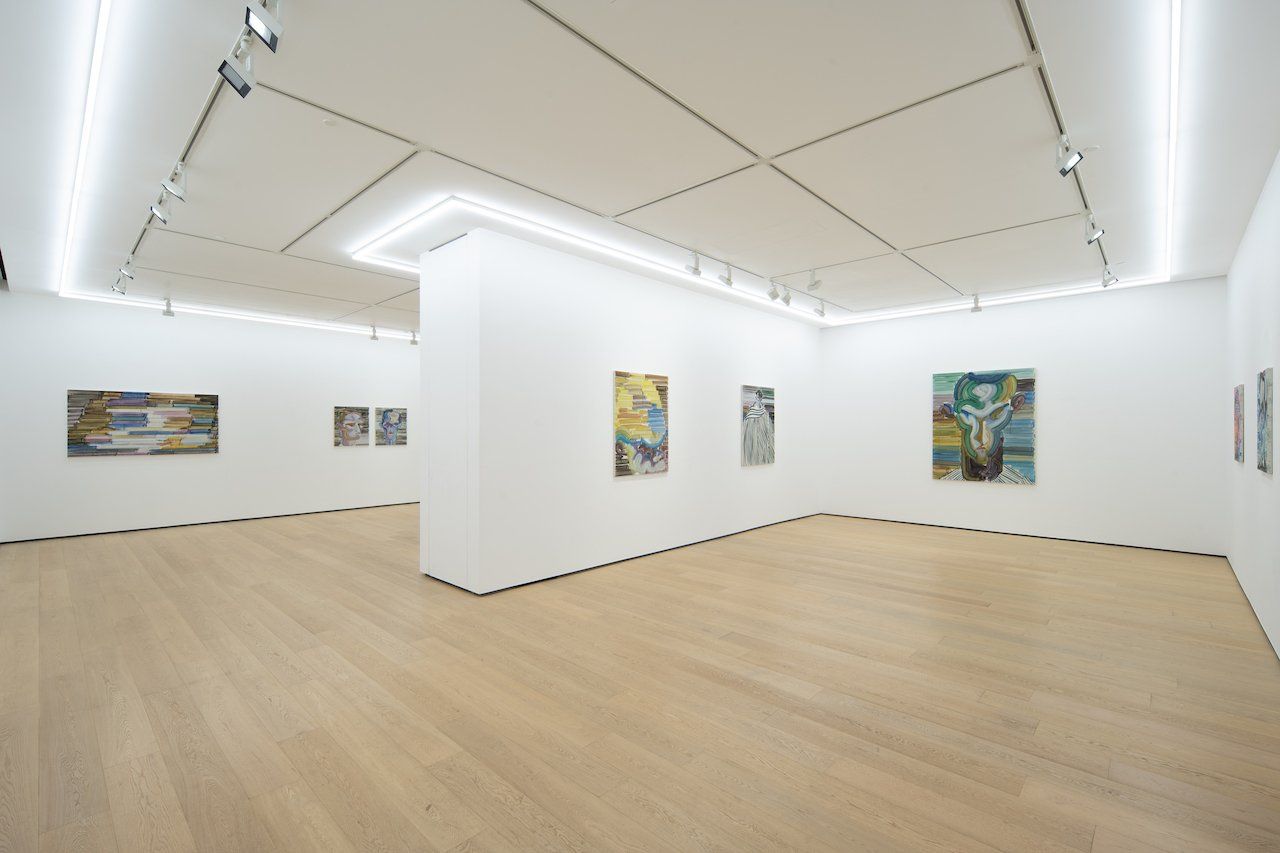The photograph depicts a clean and bright art gallery room with white walls and a light brown wooden floor. The pale wooden planks and white ceilings with panel divisions create a modern and airy aesthetic. Bright, fluorescent lighting, both in lines of individual light bulbs and LED strips around the room, ensures the space is well-lit. The gallery features a range of abstract paintings, all unframed canvases. These artworks include colorful compositions and some with discernible figures, such as stern-faced men and possibly animals, although they remain abstract. The pieces vary in size, with some big, medium, and small pieces all evenly spaced across the walls. A partial wall, which is also white, extends into the room, creating a slight division that obscures a full view of the entire space. Mounted on the ceiling, there are screens or cameras that look down towards the floor, whose function remains unclear. The gallery room is empty of people, adding to its serene and uncluttered atmosphere.